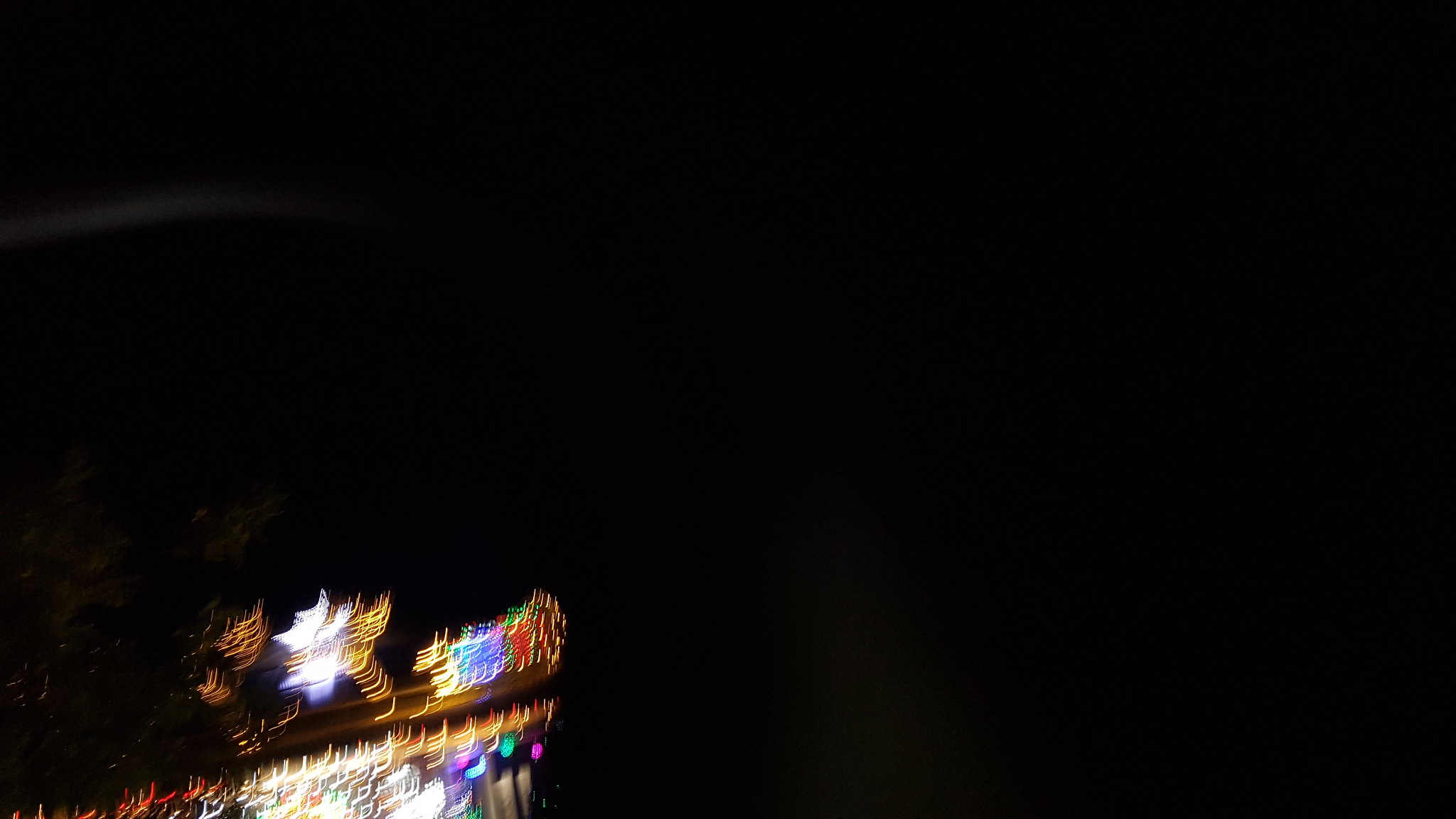This rectangular image, with dimensions twice as wide as it is tall, primarily features a black backdrop. Situated at the lower left corner, there is a highly blurred yet vividly colorful object. The object appears to be shaped like a dish, from which a square tree-like structure adorned with white lights extends upward. Complementing these lights are vibrant hues of yellow, red, and green, forming shapes akin to hockey sticks near the top. At the base, designed to resemble a Greek column, more minuscule hockey stick shapes in a variety of colors can be discerned, adding intricate detail to the piece.